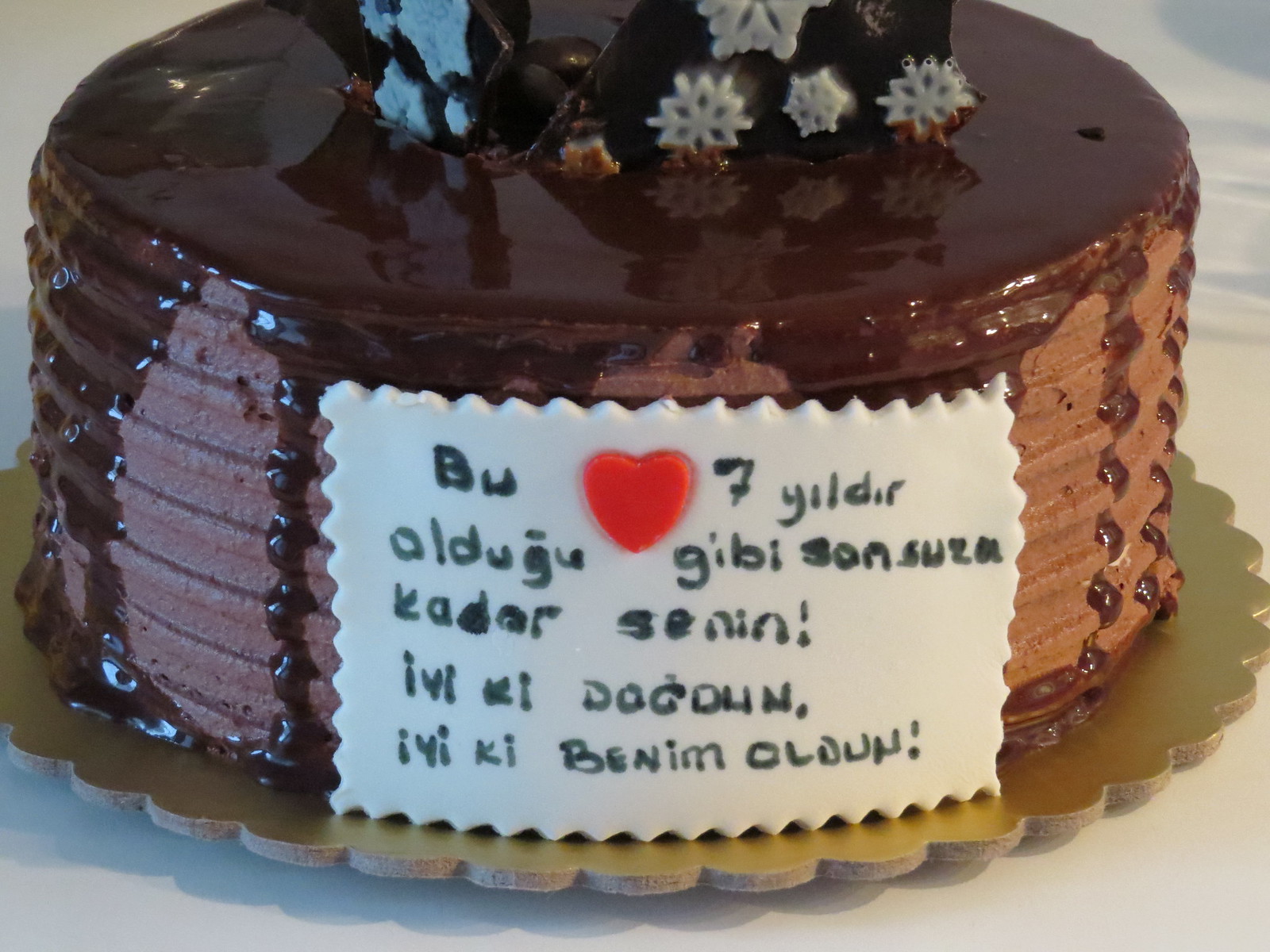This image features a close-up view of a birthday cake, composed as a slightly top-down and side perspective. The cake dominates the frame, slightly cropped at the top, showcasing a rich chocolate frosting that covers its sides, adorned with neat ridges. The surface of the cake is garnished with a glossy chocolate ganache that elegantly drips over the edges. Atop the ganache sits a decorative bow, which appears to be made of dark chocolate, accented with intricate white snowflakes.

The cake rests on a golden cake stand, likely cardboard, adding a touch of glamour to the presentation. On the front of the cake is a white fondant cutout with crimped edges, bearing a message in an unidentified language, centered around a red heart. The number "7" is included in the inscription, suggesting that this is a birthday cake. The overall presentation combines the richness of chocolate with festive winter-themed decor, making for a visually appealing and celebratory confection.